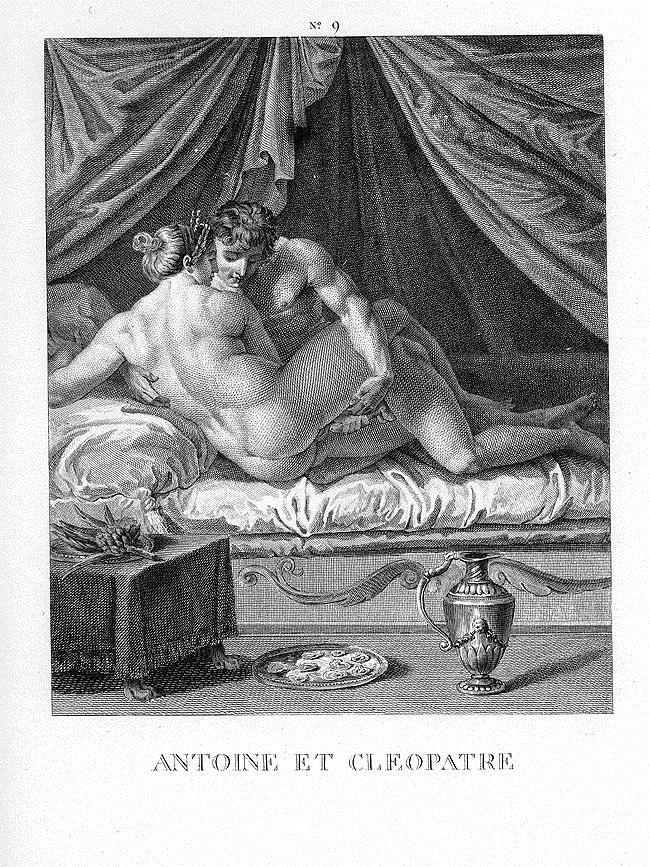This detailed, black-and-white sketch is reminiscent of Roman times and features two highly muscular figures, a man and a woman, engaged in a sexual act. Both are naked, the man positioned behind the woman, with his hands guiding her and preparing for penetration. The woman's back is turned towards the viewer, displaying her strong, defined muscles, and her hair is neatly swept up into a bun. The man, depicted with dark hair, has an equally impressive physique.

The setting is a bed with a Victorian or Roman style, adorned with numerous wrinkles on its sheet, suggesting motion and activity. Surrounding the bed are various items: a metal pitcher or urn on the floor, a plate that appears to hold oysters, and a table with a cloth draped over it, showcasing some kind of fruit. Elaborate drapes frame the background, converging in the center and cascading down the sides.

At the bottom of the image, the inscription "Antoine et Cleopatra" suggests the scene may be inspired by the legendary couple, Antony and Cleopatra. The artist used intricate detailing, possibly a technique involving dots, checks, or hatches, to create varying shades of gray, adding depth and dimension to the scene.